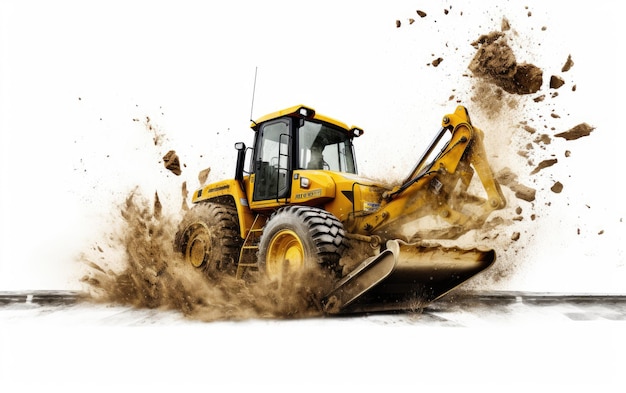The photorealistic illustration showcases a heavy-duty yellow tractor, reminiscent of Caterpillar machinery, equipped with a cab and four enormous industrial tires. The tractor is actively plowing forward, generating a dramatic scene where large clods of sandy brown dirt and rock are being forcefully thrown into the air, creating impressive smoke-like patterns of debris. The monstrous tires, particularly the rear ones, are visibly caked in mud and dirt from the intense digging action. Though the tractor’s claws are engaged in the earth-moving process, the origin of the dirt and rocks remains somewhat ambiguous. Despite the limited details of the white-on-white background, the faint silhouette of a driver is discernible within the tinted gray glass compartment, lending a human element to this robust piece of machinery.